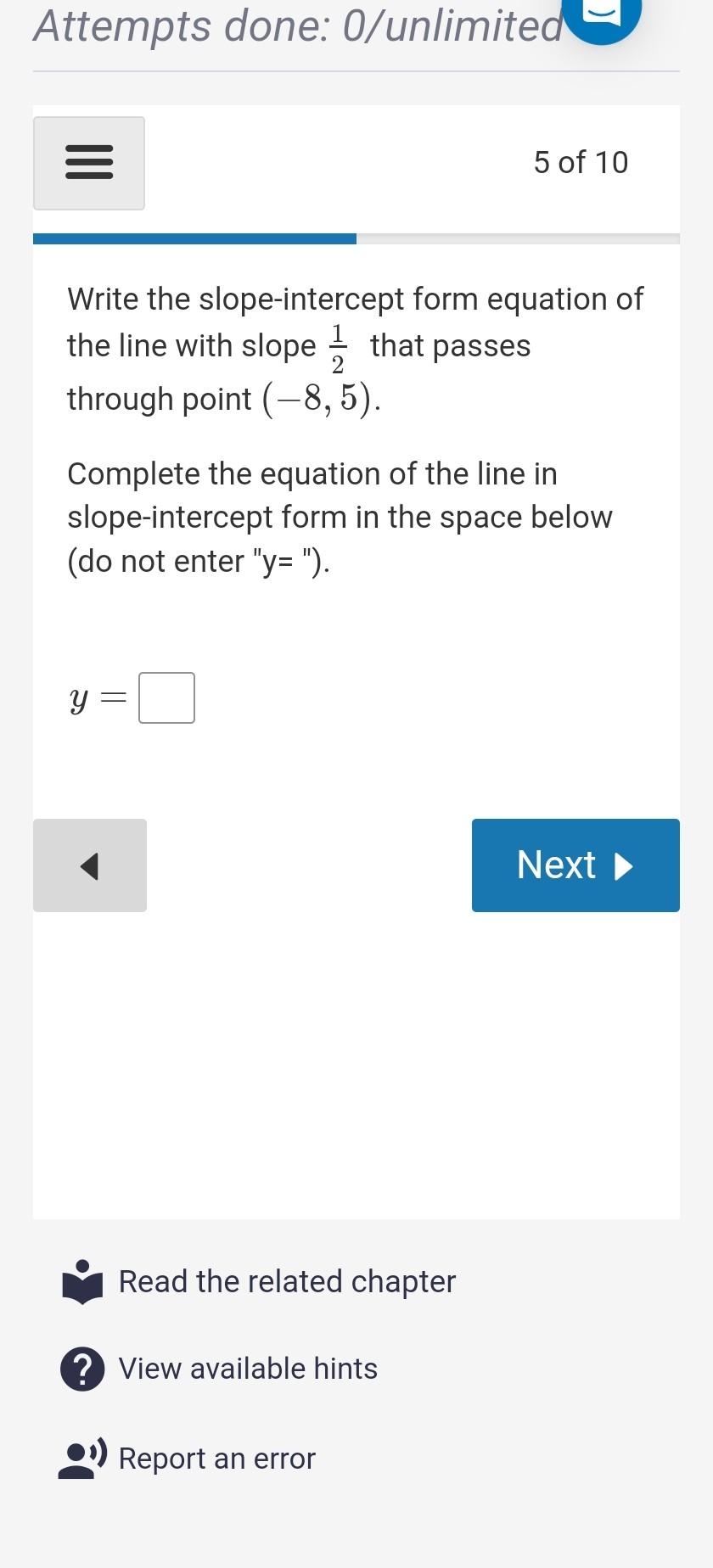The image features a multi-layered gray background with various elements arranged in a structured format. At the top, the text "Attempted: 0 / Unlimited" is prominently displayed in a muted gray color. Below this text, a horizontal gray line separates the header from the main content area.

The main section consists of a white rectangular box, which is oriented horizontally. On the left side of this box, a gray button with three black bars indicates a menu option. To the right, the text "5 of 10" is displayed, denoting the progress of an activity.

Beneath this, a progress bar is shown, with its left half filled in blue and the right half in gray, representing partial completion.

Further down, there is a vertically oriented red and white rectangle containing an instructional text in black. The text reads: "Write the slope/intercept form equivalent equation of the line with the slope of 1/2 that passes through the point (-8, 5). Complete the equation of the line in the slope-intercept form in the space below (Do not enter 'y =')."

Following this instruction, the text "y =" is displayed next to a white input box outlined in black, where the user is expected to enter their equation. 

At the bottom, there are two buttons: a gray button with a black left-pointing arrow on the left, and a blue button labeled "Next" in white text on the right, suggesting navigation options.